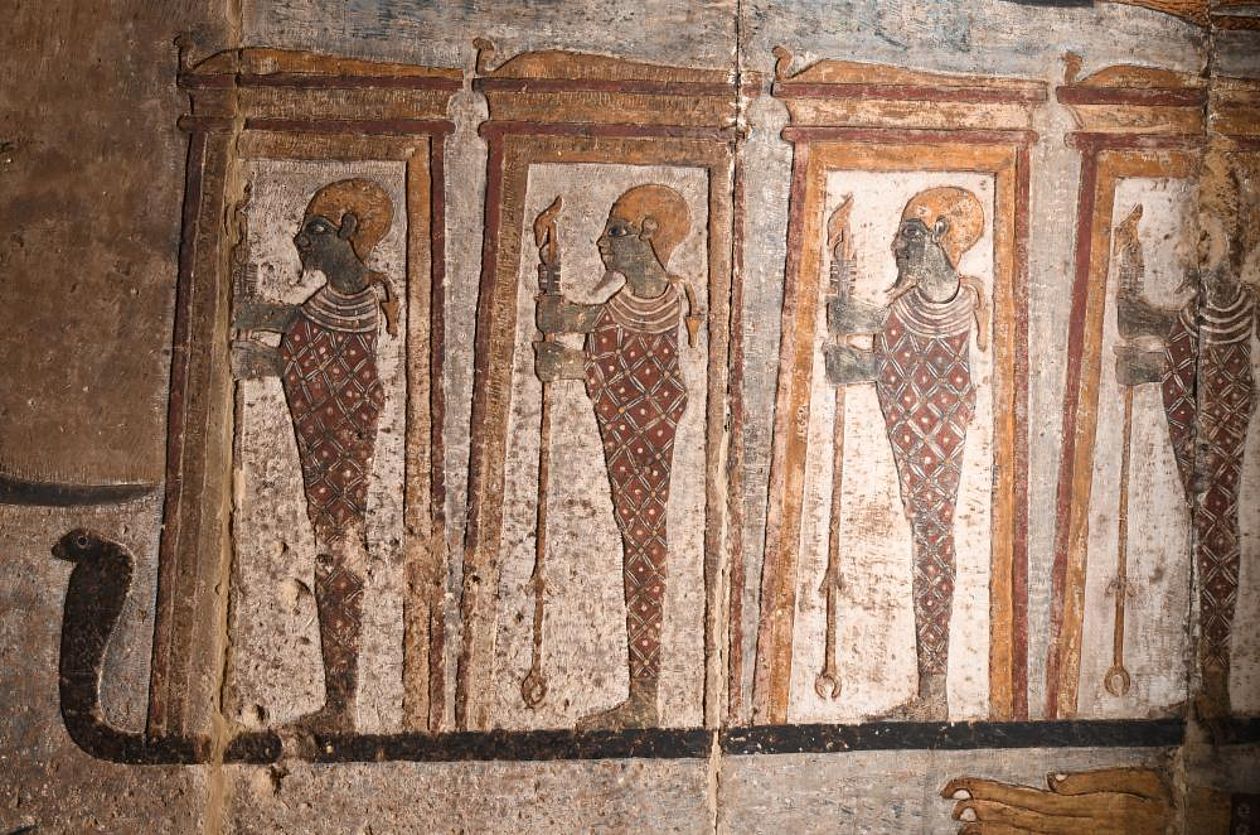The photograph captures an intricate piece of ancient Egyptian artwork carved and painted onto a stone wall. Vivid colors of gold, red, black, and some browns dominate the composition. The scene depicts four identical, black-skinned figures clad in red robes with diamond patterns, holding golden scepters or staves. They stand in profile, facing left, within what looks like doorways or telephone box-shaped structures. These figures are positioned on the back of a long snake that stretches horizontally across the image. The snake's body curves up into a flared cobra head on the left side of the image. There is no text, other animals, buildings, or modern elements present in the image, which focuses entirely on the ancient artistry and the depicted figures.